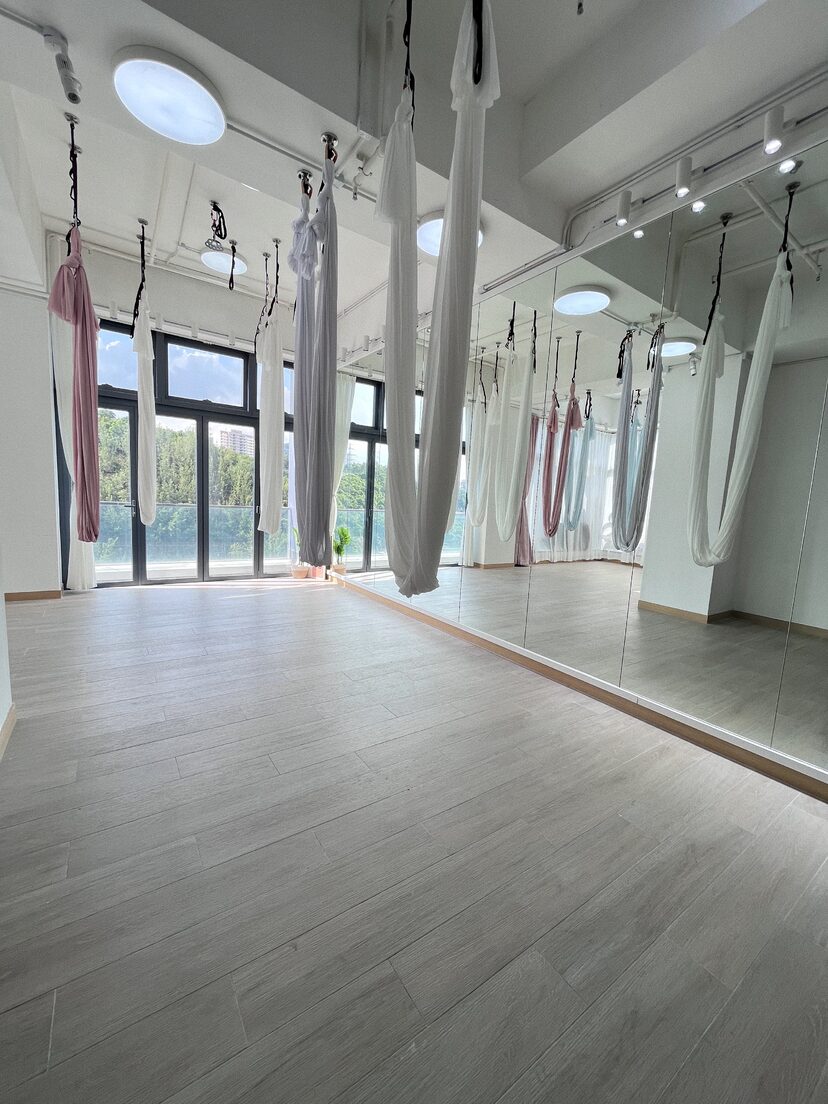This photograph captures the interior of a spacious and empty dance studio with a distinctive grayish wooden plank floor. The right side of the studio features a floor-to-ceiling wall of tall rectangular mirrors, bordered at the bottom by a strip of brown molding. On the opposite side, large glass double doors open onto a small balcony, offering a view of lush green foliage and blue skies beyond. The ceiling is painted white and dotted with both large and small lights, illuminating the space below. Suspended from the ceiling are several thick and sturdy U-shaped fabric strips in red, white, and gray, attached at two points by black cords. These fabrics resemble those used in acrobatic or aerial performances, often seen in Cirque du Soleil performances, suggesting this studio might be used for such forms of dance or aerial arts.